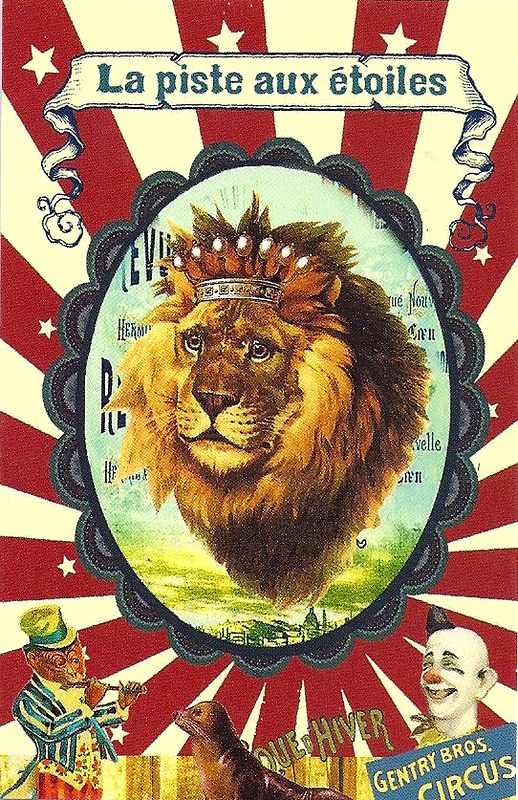The vibrant vintage circus poster features a primarily red, white, and blue color scheme with a white background adorned by red stripes radiating from a central point. At this focal point is an illustration of a male lion's head crowned regally, evoking a sense of grandeur. Above the lion, a banner displays the French words "La Piste aux Étoiles," enhancing the allure. The bottom of the poster is lively with a clown in the bottom right corner, characterized by his red nose and small black hat, holding a sign that reads "Gentry Brothers Circus." To the left of the clown, a monkey dressed in a striped suit and top hat is playing a flute, accompanied by a seal nearby gazing at the monkey. The overall design is a nostalgic tribute to classic circus advertisements.